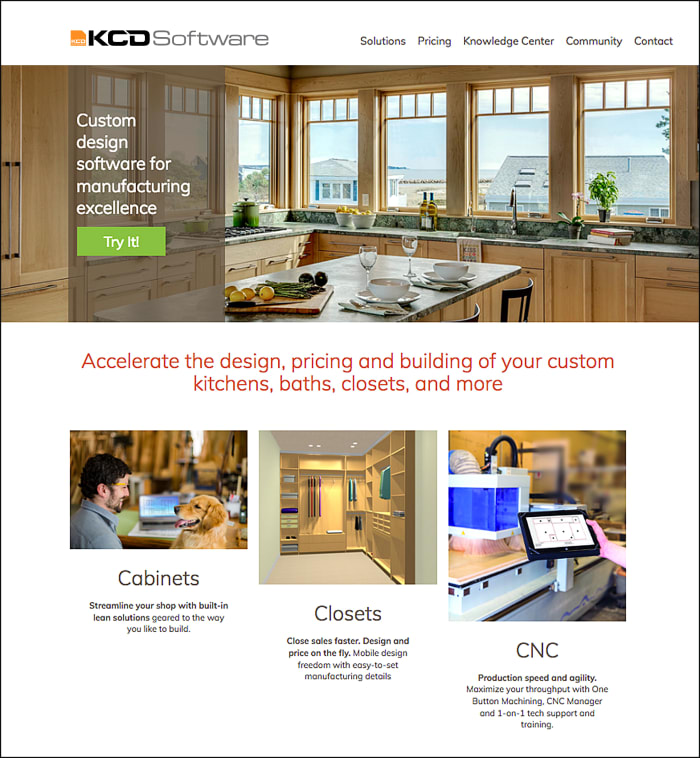This image is taken from the KCD Software website. At the top of the page, a navigation menu featuring the options "Solutions," "Pricing," "Knowledge Center," "Community," and "Contact" extends towards the right.

In the middle section of the image, a well-appointed kitchen counter is prominently displayed. The counter is set with plates and bowls prepared for food, and a cutting board holds fresh asparagus and lemons. The kitchen is flooded with natural light from numerous windows encircling the space. Below this scene, a bold red caption reads: "Accelerate the design, pricing, and building of your custom kitchens, baths, closets, and more."

Continuing downwards, the lower section of the image features a man joyfully smiling at a golden retriever. In the background, a computer is visible. The section is dedicated to different features offered by KCD Software. It includes:
- Cabinets: "Streamline your shop with built-in lean solutions geared to the way you like to build."
- Closets: "Close sales faster, design and price on the fly, mobile design freedom with easy-to-set manufacturing details."
- A brief paragraph under the label "CNN."

Overall, the image composition effectively showcases the user-friendly interface and versatile functionalities of the KCD Software, highlighting its capabilities in custom kitchen design and more.